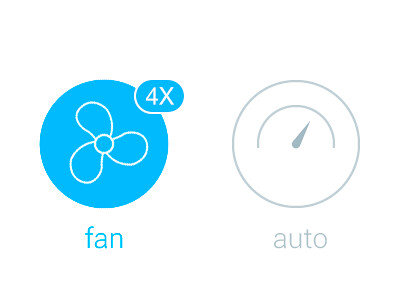The image is a simple illustration with a white or transparent background, featuring two identically sized circles side by side. The circle on the left is a solid turquoise or sky blue with a white outline of three curvy fan blades centered inside, indicating a fan. Attached to the top right of this blue circle is a blue oval with "4X" written in white lettering. Beneath the blue circle, the word "fan" is written in matching blue font.

To the right, there is a grey-outlined circle with a thin grey line. Within this circle, starting from the middle left and arcing to the middle right, is a semi-circle arc containing a small pointer dial. Below this grey-outlined circle, the word "auto" is written in grey lowercase letters.